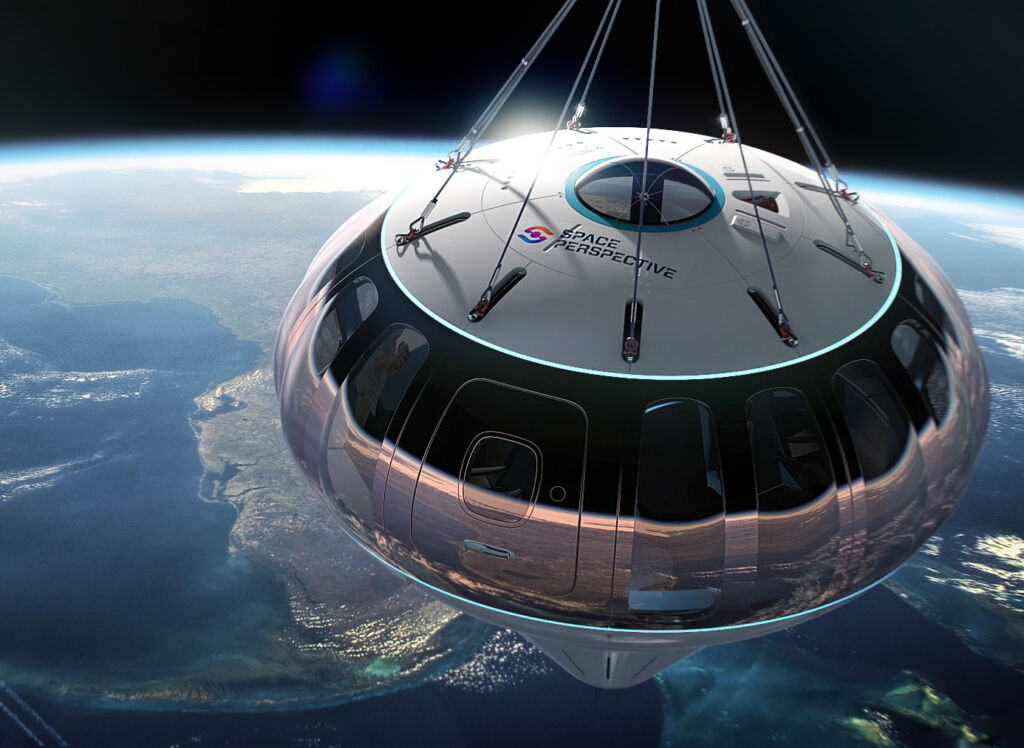The image, a digitally-rendered scene set in the vastness of outer space, showcases a uniquely designed spaceship resembling a large, shiny half-sphere with a conical white base. This spacecraft, positioned in the upper right corner of the image, appears to be floating or descending in space. Its reflective surface mirrors the planet below, displaying an aerial view of Earth’s blue oceans, green continents, and swirling white clouds. The spaceship features multiple windows and an observation deck inside, as indicated by the numerous windows allowing an unobstructed view of the planet. The spacecraft’s side prominently displays the text "Space Perspective" and an accompanying logo with a stylized letter "S" incorporating a red dot in its center. Supporting the vessel are multiple metal wires converging at a single point above it, potentially connecting to a parachute system. The background transitions from a black expanse of outer space at the top to the bluish-gray and white hues of Earth dominating the bottom portion, emphasizing the vessel’s position in the vast void between the two realms.